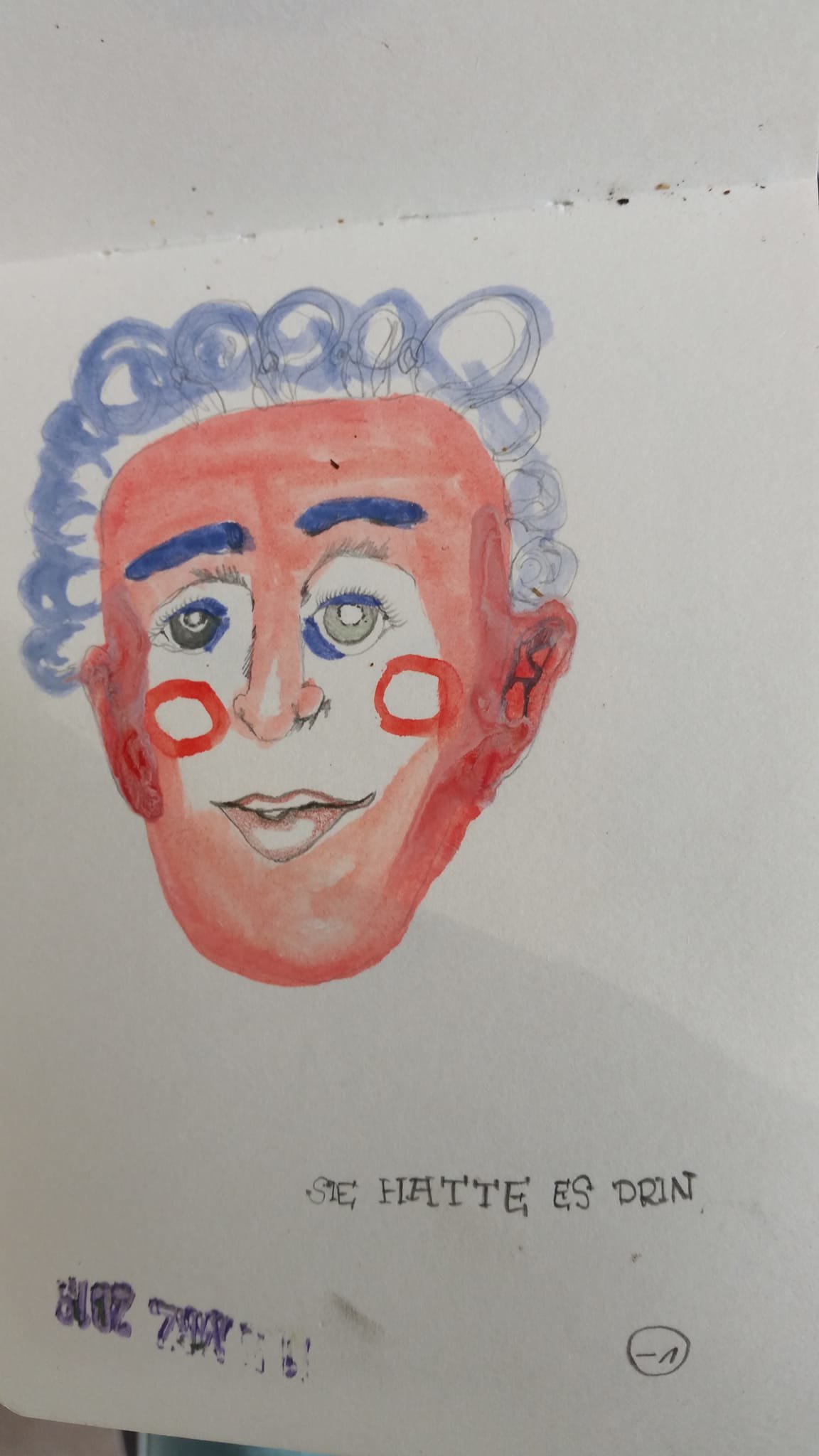This artwork is an expressive illustration or painting, created on a stark white sheet of paper. The piece features a stylized portrait drawn with pen or pencil, and enhanced with vibrant paint. The subject of the portrait is a face with striking, curly blue hair, complemented by dark blue eyebrows and a subtle touch of blue eyeliner. The face is predominantly painted in a vivid red, except for the central area around the nose, eyes, and upper lip, which remains white. This contrast, along with the red circles adorning both cheeks, gives the portrayal a clown-like appearance, reminiscent of theatrical face paint. Beneath the vividly depicted face, a small inscription reads, "Hattie as Dren." The exact text is somewhat unclear, but it unmistakably consists of words, adding a layer of intrigue to the piece.